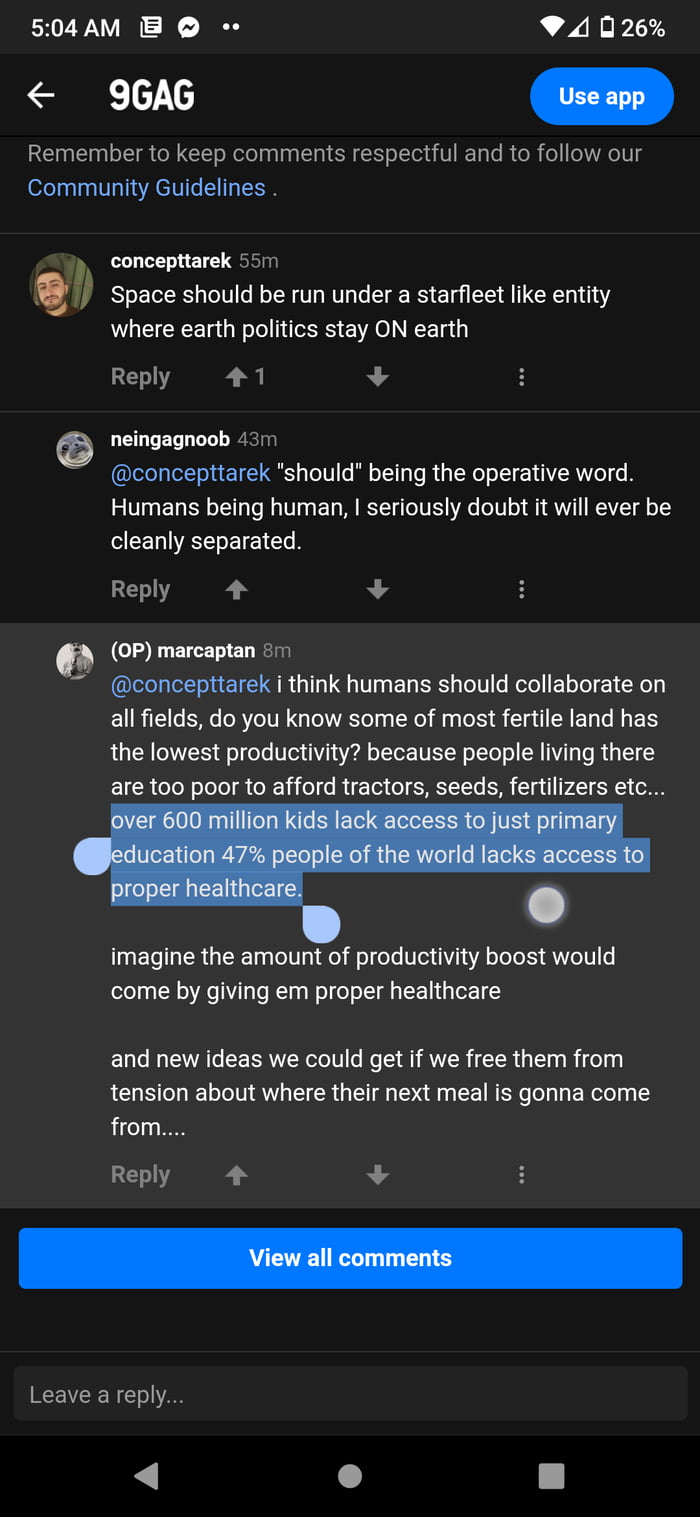Screenshot Description:

The screenshot features a user interface with a black background. At the top, the time is displayed as 5:04, and the battery level is at 26%. The screen includes text in blue with a clear reminder to keep comments respectful and to follow the community guidelines.

A blue oval button prompts users to "Use app." Below, there are multiple profile pictures and comments. 

1. The first comment is from a user with a profile picture of God. This comment, posted 55 minutes ago, discusses a hypothetical scenario where a spaceship is operated under a Starfleet-like entity, implying that Earth politics should remain on Earth. There are buttons to reply, an up arrow with a count of 1, a down arrow, and three vertical dots for more options.

2. The second comment features a profile picture of what appears to be a panda, posted 43 minutes ago by a user named Tariq (T-A-R-E-K). The comment is in quotations and discusses the difficulties in cleanly separating human behaviors due to inherent flaws, with "should" being emphasized. As with the first comment, there are options to reply, an up arrow, a down arrow, and three vertical dots for additional actions.

3. The third visible comment has a profile picture of a man and was posted 8 minutes ago. Similar interaction options—reply, up arrow, down arrow, and three vertical dots—are available.

This structured layout helps in keeping track of comment timelines, interactions, and user profiles within the application.